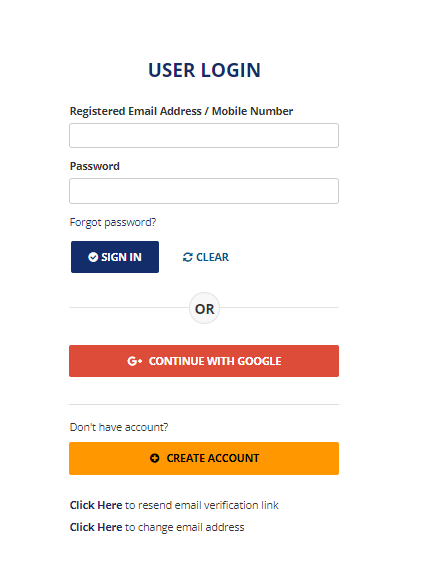The image depicts a user login interface for a website. At the very top center, the header reads "User Login" in blue text. Below this header, there are two primary input fields. The first field, labeled "Registered Email Address/Mobile Number," is currently empty. Directly beneath it, the second field is labeled "Password" and is also empty.

Underneath the password field, there is a "Forgot Password" link displayed in light blue text. Moving further down, there are two buttons side-by-side. The left button is blue, with the text "Sign In" in white, accompanied by a checkmark icon. The button on the right is blue and labeled "Clear," featuring an icon of a circular arrow indicating a reset or refresh action. 

Additionally, the section is visually separated by a horizontal gray line with the word "or" centered within a gray circle, flanked by short gray lines. Below this separator, there is a prominent red button labeled "Continue with Google," featuring Google's "G" icon to the left.

Following another gray horizontal separator, a message reads "Don't have an account?" This is accompanied by an orange button labeled "Create Account" in black text, accentuated with a plus icon. At the very bottom of the interface, there are two more clickable options: "Click here to reset email verification link" and "Click here to change email address."